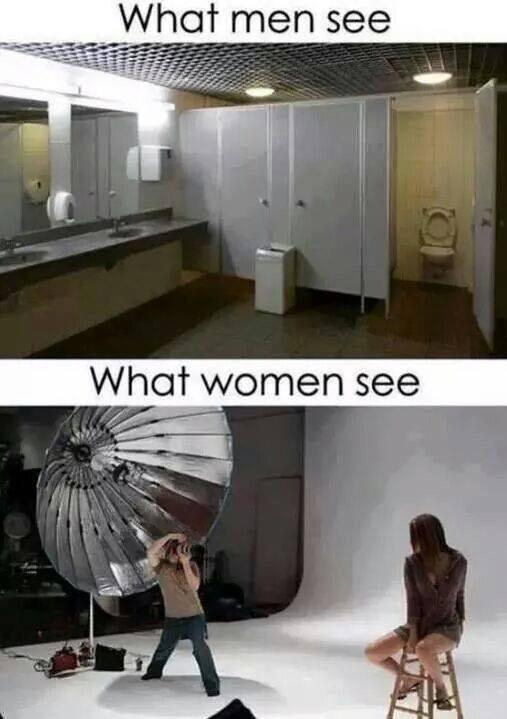The image is split into two stacked photographs, creating a contrast between two different scenes. The top photograph, titled "What Men See," depicts an empty bathroom. It features three stalls, one of which is open, exposing a toilet. There's also a trash can, a soap dispenser, a sink, and mirrors visible to the left. The color palette includes shades of black, white, brown, tan, gray, yellow, blue, and red, lending a typical utilitarian look to the bathroom.

The bottom photograph, labeled "What Women See," depicts a commercial photography setting. In this scene, a female model with dark hair, wearing shorts, is seated and leaning forward on a stool. A photographer is kneeling on the floor, aiming his camera at her, with a large steel reflector positioned behind him to enhance the lighting. Both scenes are presented in a photographic realism style and are likely arranged as a meme intended for social media sharing on platforms like Facebook or Twitter.